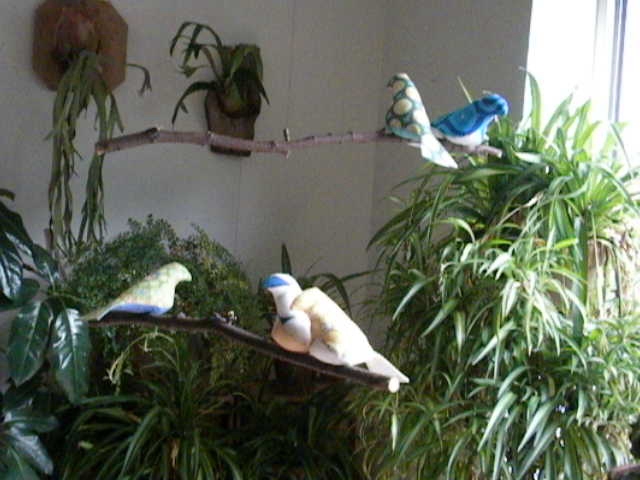This is a detailed color photo taken indoors, likely within a house or an apartment with white paneled walls and a window on the right side that allows sunshine to brighten the room. The room is densely adorned with various green plants, creating a lush, greenhouse-like atmosphere. On the right side of the photo, amidst the green, long leaves, a sturdy horizontal brown branch stretches across the image, supporting two vibrantly colored birds. These birds, likely artificial and resembling bean bags or hacky sacks in texture, display a vivid combination of blue, green, and yellow with long tails. Towards the left side of the scene, another brown branch lies lower down, closer to the viewer, hosting two more similar decorative birds. These birds exhibit an array of unusual colors: one is lime green, while the other displays a mix of blue shades, green with yellow circles, and another with white, yellow, and blue accents. The leafy plants in the room vary in type, with some hanging on the walls and others more shrub-like, contributing to the overwhelmingly verdant decor of this intriguing interior space.